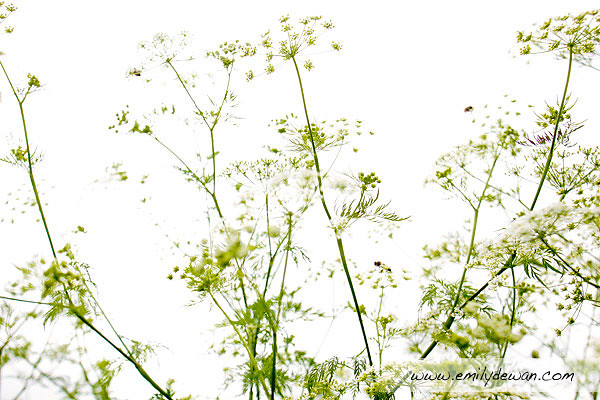The image features a bright white background, creating the impression of an outdoor setting under intense daylight. Central to the composition are several delicate plants, their thin green stems adorned with clumps of flower buds. The buds, resembling small bursts of green interspersed with hints of white and possibly yellow, evoke a likeness to Queen Anne's lace. These floral clusters, typically in groups of three or four, are scattered across the center, right, and left portions of the image, blending seamlessly with the luminous background. In the bottom right corner, a website URL, www.emilydewan.com, is subtly inscribed in black, adding a touch of informational detail without detracting from the natural beauty of the scene.